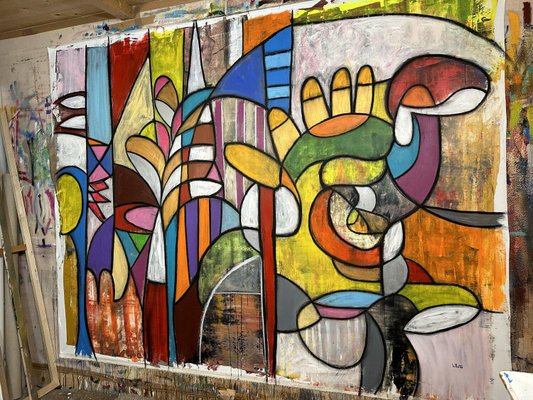This vibrant piece of artwork appears to be a graffiti-style mural, possibly painted or spray-painted on a street canvas. The rectangular canvas was originally white but is now a vivid explosion of abstract shapes and designs, primarily round, including ovals, orbs, and disks. The mural is partitioned into various sections and enveloped by a subtle white border. Within the artwork, there is a prominent, multicolored hand, featuring shades of yellow, orange, green, red, purple, and blue. This hand adds a unique layer of intrigue to the overall abstract composition. The vivid palette includes striking hues of black, gray, brown, various blues, violet, pink, yellow, red, and stripes of orange and purple, enhancing the artwork's dynamic and chaotic appeal. Amidst the colorful chaos, elements such as striped sections and yellow finger-like shapes stand out, though the mural remains dominantly abstract with no text. Bursting with vibrant colors and unique patterns, this mesmerizing artwork forms an intriguing tapestry of modern street art.